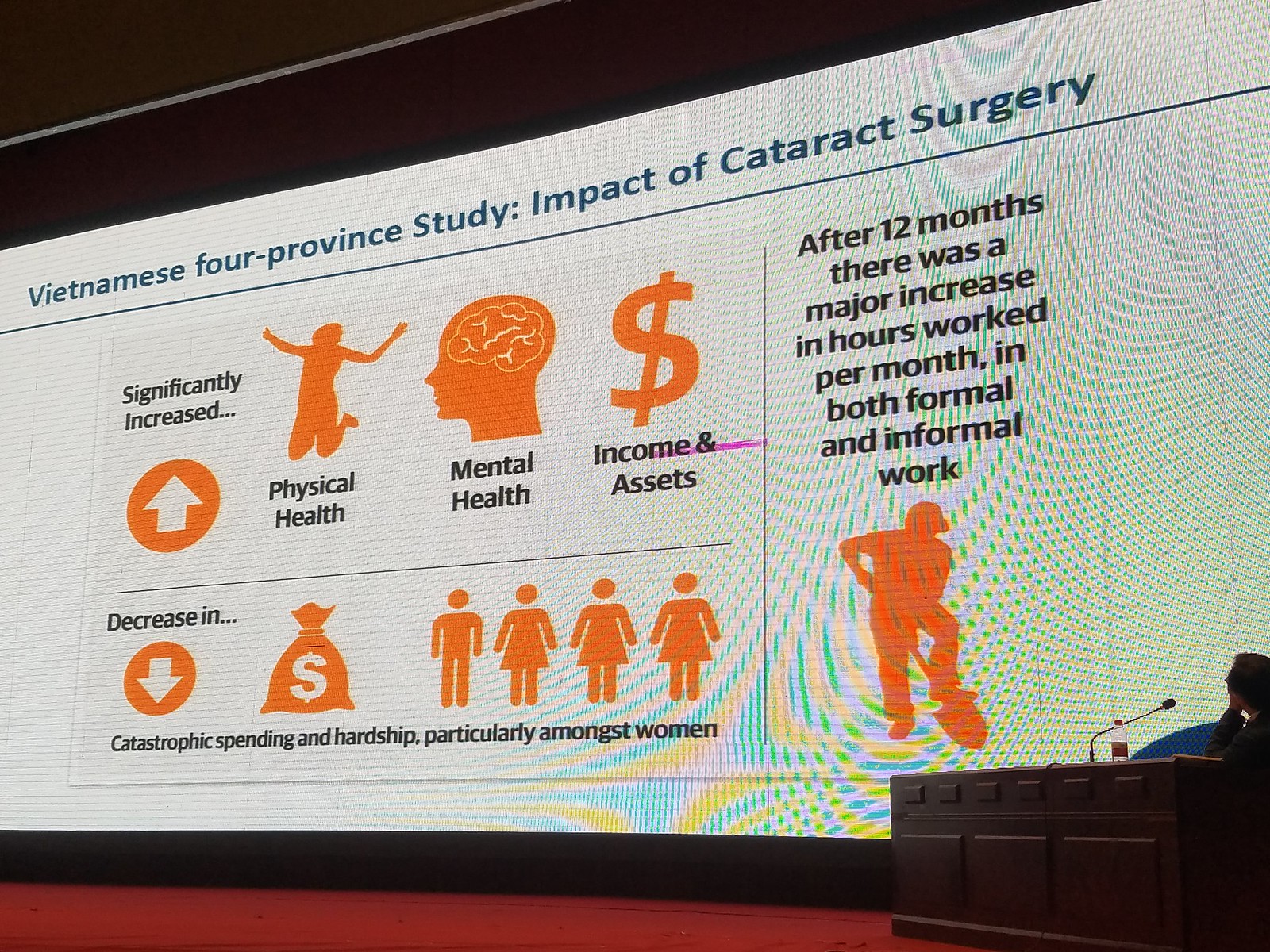This photo captures a scene from a presentation on a stage with red carpeting. Positioned on the right side, a solid wooden desk holds a microphone in the center and a bottle of water, with a person sitting behind it, facing away from the camera and towards a large projected screen. The screen displays a detailed slide titled "Vietnamese Four Province Study Impact of Cataract Surgery." 

This presentation highlights significant findings, including a notable increase in physical health, mental health, and income and assets, illustrated with specific icons: a silhouette of a person jumping (physical health), a head with a lit-up brain (mental health), and a dollar sign (income and assets). Additionally, a white arrow inside an orange circle signifies the upward trend of these improvements. Below, it is mentioned that there is a decrease in catastrophic spending and hardship, particularly among women, represented by a money bag and figures of one male and three females, with a white downward-pointing arrow in an orange circle indicating the decline. 

On the right side of the slide, it details that after 12 months of cataract surgery, there was a significant increase in the number of hours worked per month in both formal and informal sectors, showcasing the broader economic benefits of the surgery.